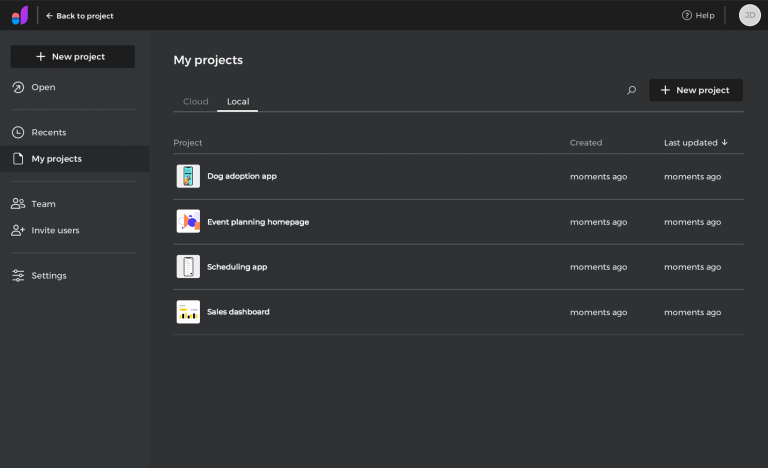The image showcases a user interface against a black background. In the top left corner, there's a small square featuring a purple line at the top. Below the line, there are two semi-circles—one red and one blue. Adjacent to this is a white arrow pointing to the left with the text "Back to Project." To the right, there's a small circle containing a question mark labeled "Help." Next to it is a line followed by a white circle with the number "20" inside.

Below this header is a button labeled "Plus New Project." The interface also includes various options such as "Open," "Recents," "My Projects," "Team," "Invite Users," and "Settings."

In the middle section, under "My Projects," the interface lists projects categorized as "Local." The project names include "Dog Adoption App," "Event Planning Homepage," "Scheduling App," and "Sales Dashboard."

On the right side, a section labeled "New Project" displays the project creation status. It lists the creation and last updated timestamps, which say "Moments ago," repeated eight times down this column.